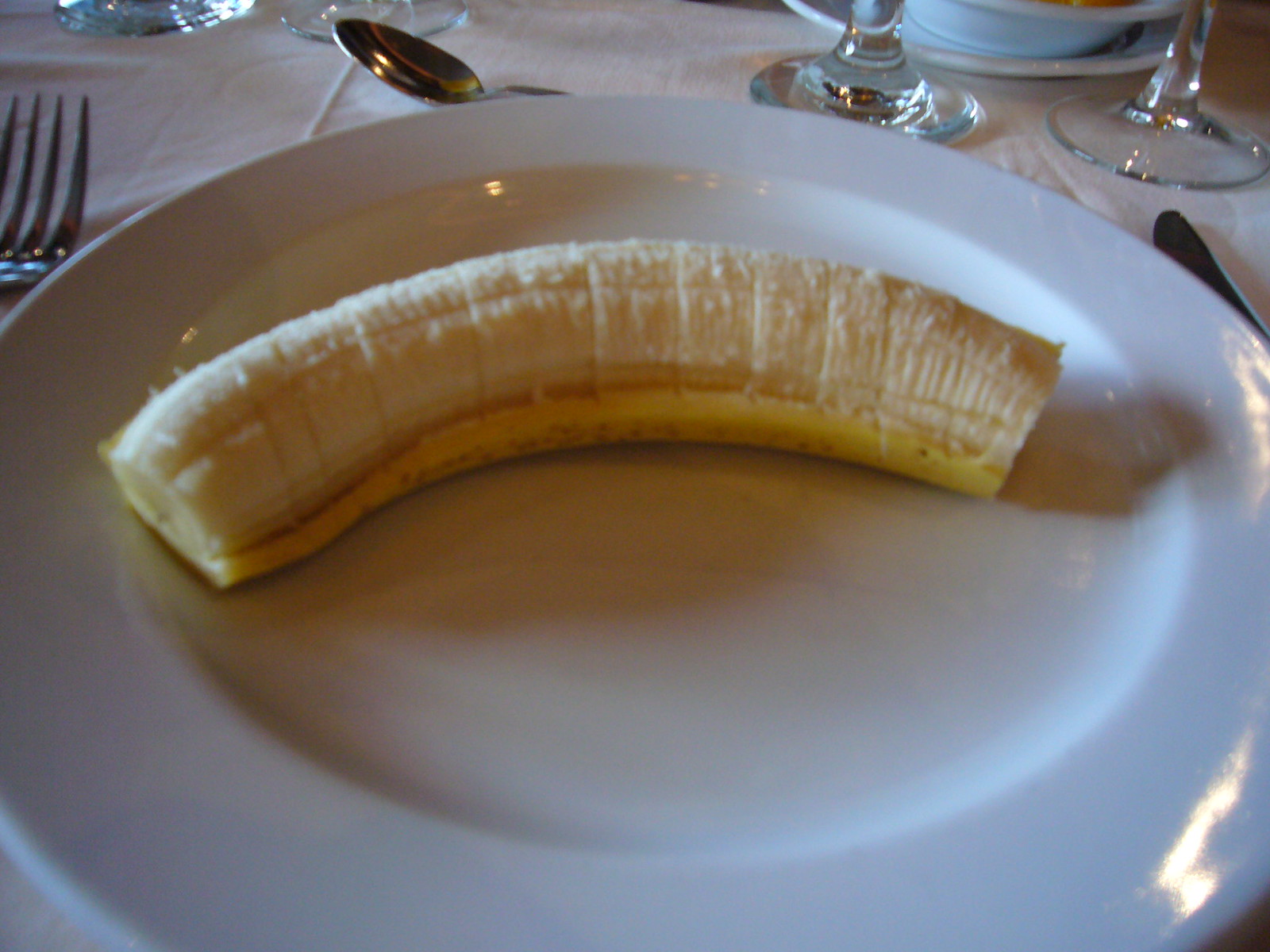The photograph features a peeled banana artfully displayed on a round white porcelain plate. The image is rectangular, with the longer sides at the top and bottom, and it is taken at an angle that causes the bottom edge of the plate to appear blurry and larger. At the center of the plate, which has a slight round recess, lies a yellow oblong banana with both pointed ends neatly trimmed off. The banana is positioned with its curved side facing upwards, directed towards the top of the plate.

The plate itself rests on a flat table draped with a white fabric tablecloth, which has several noticeable folds and wrinkles. On the right side of the plate, partially tucked under its lip, is a dull silver-colored butter knife. A matching four-prong silver fork is also placed slightly underneath the lip to the right. Above the plate, positioned sideways, is a silver spoon with its head pointing towards the left side of the image.

In the background, multiple stems of glasses can be seen towards the top right and left corners of the image, adding a touch of elegance. Additionally, a white porcelain bowl is visible in the top right corner, complementing the setting.